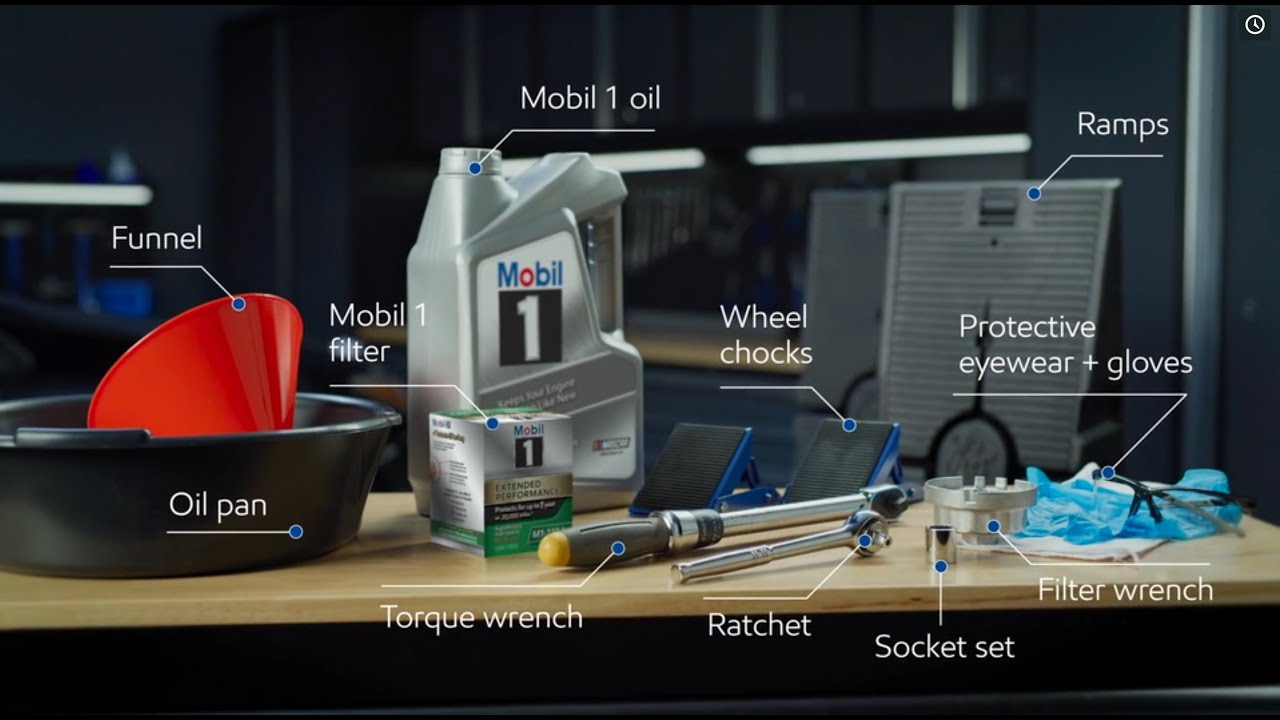This is a close-up, indoor color photograph of a workbench showcasing a detailed collection of tools essential for an oil change, each labeled with white text and arrows pointing to the respective items. From left to right, the meticulously arranged items include a black oil pan with a red funnel inside labeled "funnel," a large container of Mobil 1 oil, and a Mobil 1 oil filter still in its box. A black-handled torque wrench with a yellow end is placed next to a chromed ratchet in the foreground. The photograph also includes a socket set, a filter wrench labeled as "oil filter wrench," blue protective gloves with a pair of safety glasses placed on top, and a set of wheel chocks. In the background, partially obscured against the predominantly dark setting, are automotive ramps. All these items rest on a tannish brown workbench, providing a comprehensive visual guide for an oil change setup.